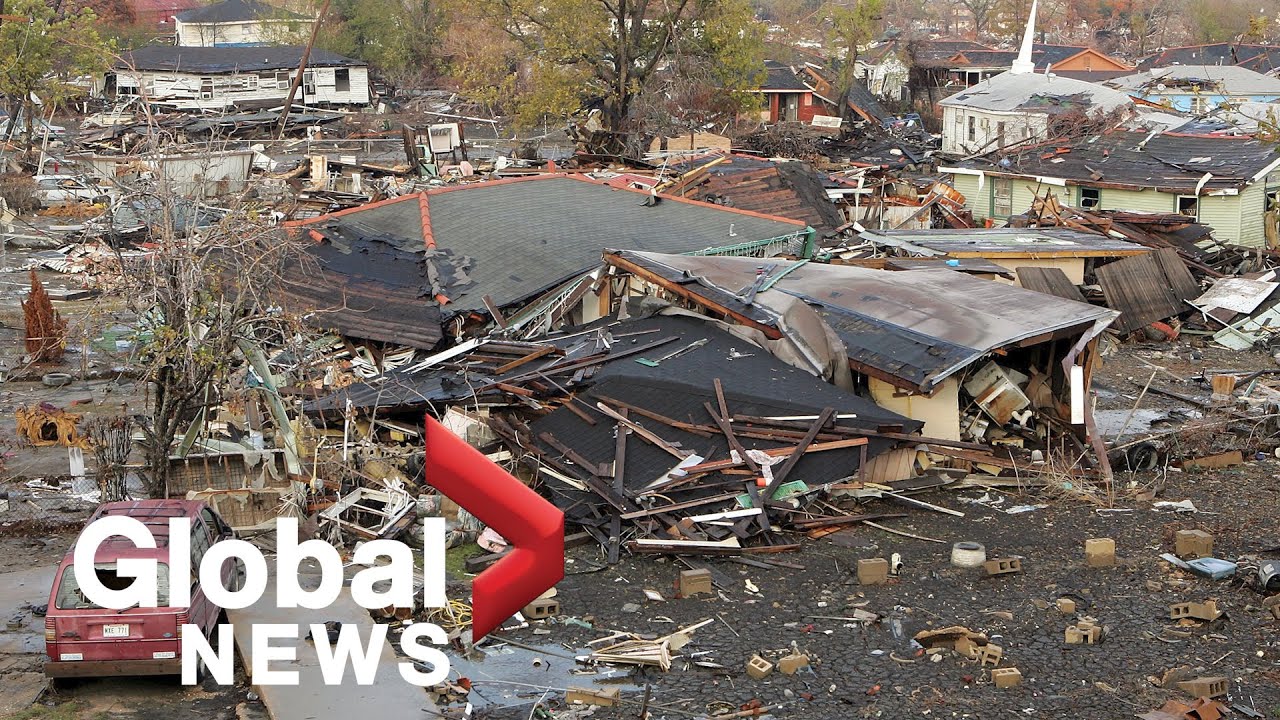The image captures the devastating aftermath of a tornado in a town. In the bottom left corner, the logo for Global News is prominently displayed with white text and a distinctive red arrow design. The scene reveals the extensive destruction caused by the tornado: buildings lie in ruin with debris, such as wood, bricks, and roof materials, scattered across the wet, darkened ground. The foreground features a red car with broken windows, emphasizing the violence of the storm. Among the wreckage are various homes and a notable white church with a gray, damaged roof and an intact steeple. The desolate area is devoid of people, highlighting the severity of the disaster. Amidst the destruction, trees are shown broken and leafless, although some in the background retain their foliage. The image powerfully conveys the chaos and devastation wrought by the tornado, making it a significant news scene.